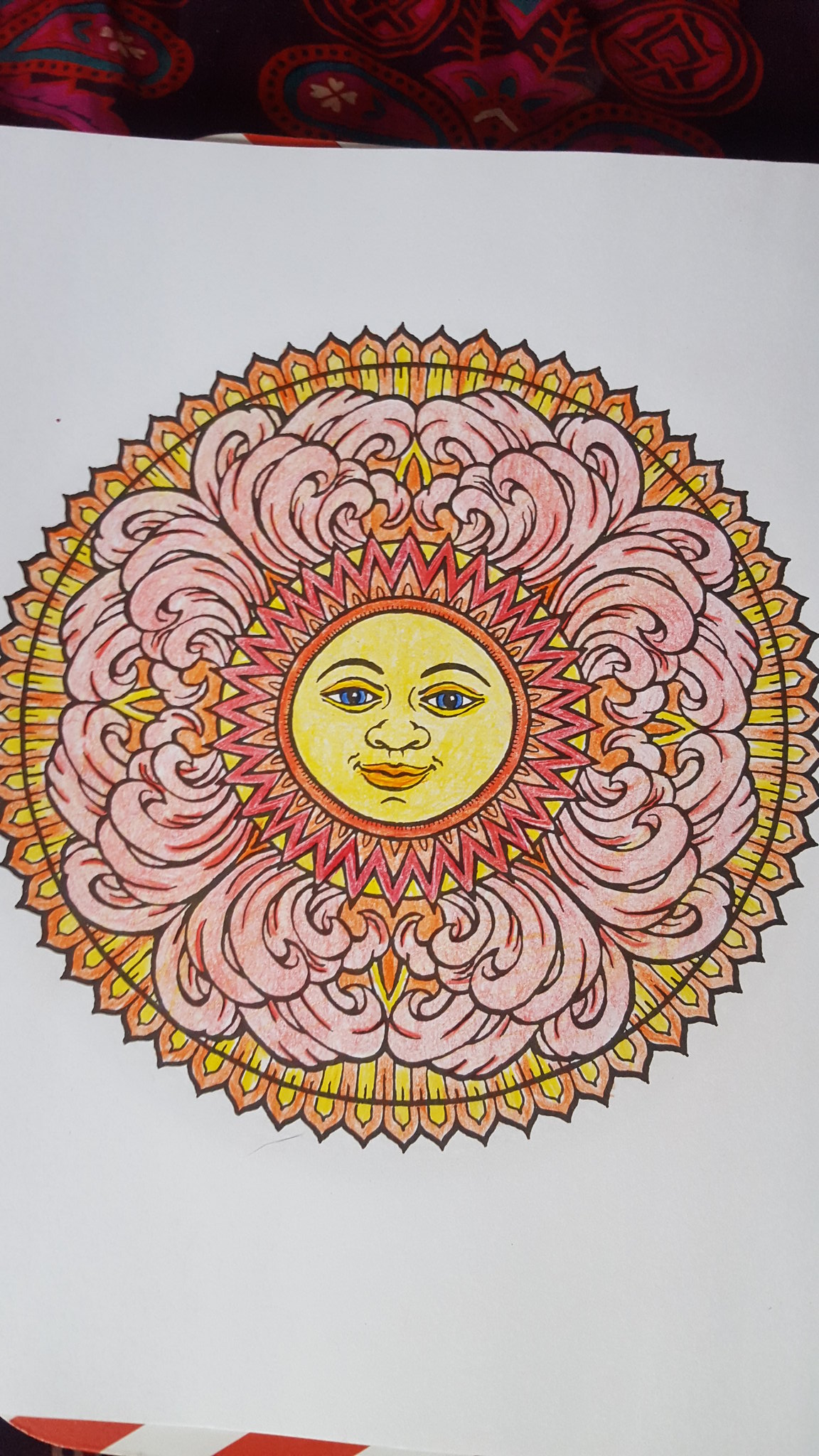This image showcases a vibrant, circular art drawing that elegantly represents the sun. At the center of the composition is a yellow face, symbolizing the sun's radiant presence. Surrounding this central face are intricate, curly feather-like designs rendered in pink, giving a sense of dynamic movement and decorative flair. Extending beyond the feathers are sharp, pointed elements in hues of yellow and orange, highlighted by precise black line work that adds depth and detail. The personified sun face features orange lips, further enhancing its vivid character. All of this stunning artistry is set against a crisp white background, allowing the bright colors to stand out beautifully.